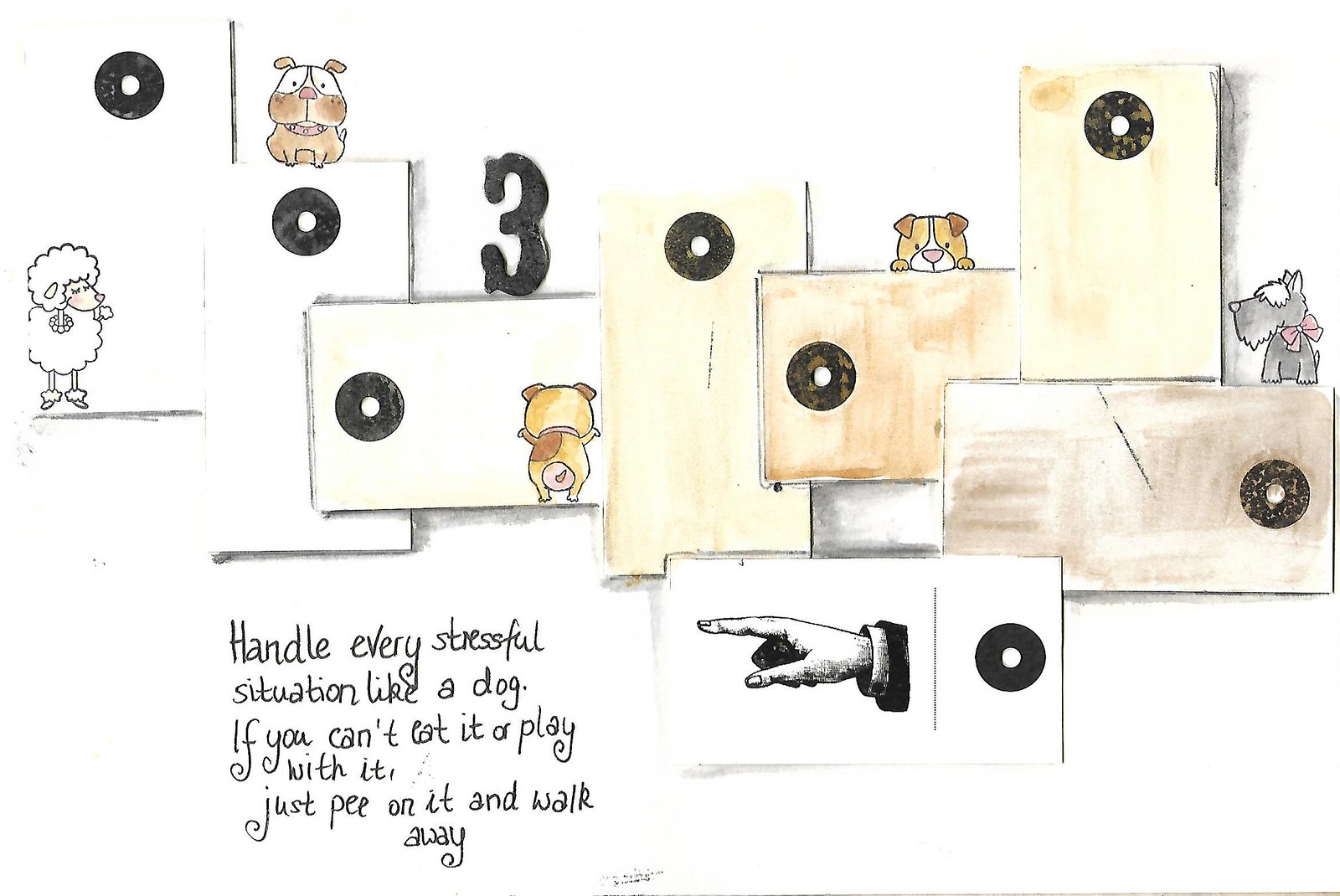In this artistic image, several hand-drawn objects are scattered, each uniquely contributing to the overall composition. On the left side of the frame, we see a thoughtfully illustrated sheep. Surrounding the sheep, there are four distinct depictions of dogs, each varying slightly in posture and expression. The dogs are rendered in contrasting shades of black, white, gray, tan, and brown. Among these images, there is also a drawing of a hand pointing to the left, likely symbolizing a direction or guidance. The composition is intentionally uncentered and disordered, suggesting a casual, freeform artistic approach. At the base of the image, a humorous and positive message reads: "Handle every stressful situation like a dog. If you can't eat it or play with it, just pee on it and walk away." This statement highlights the lighthearted and whimsical nature of the artwork, offering a playful philosophy towards handling life's challenges.